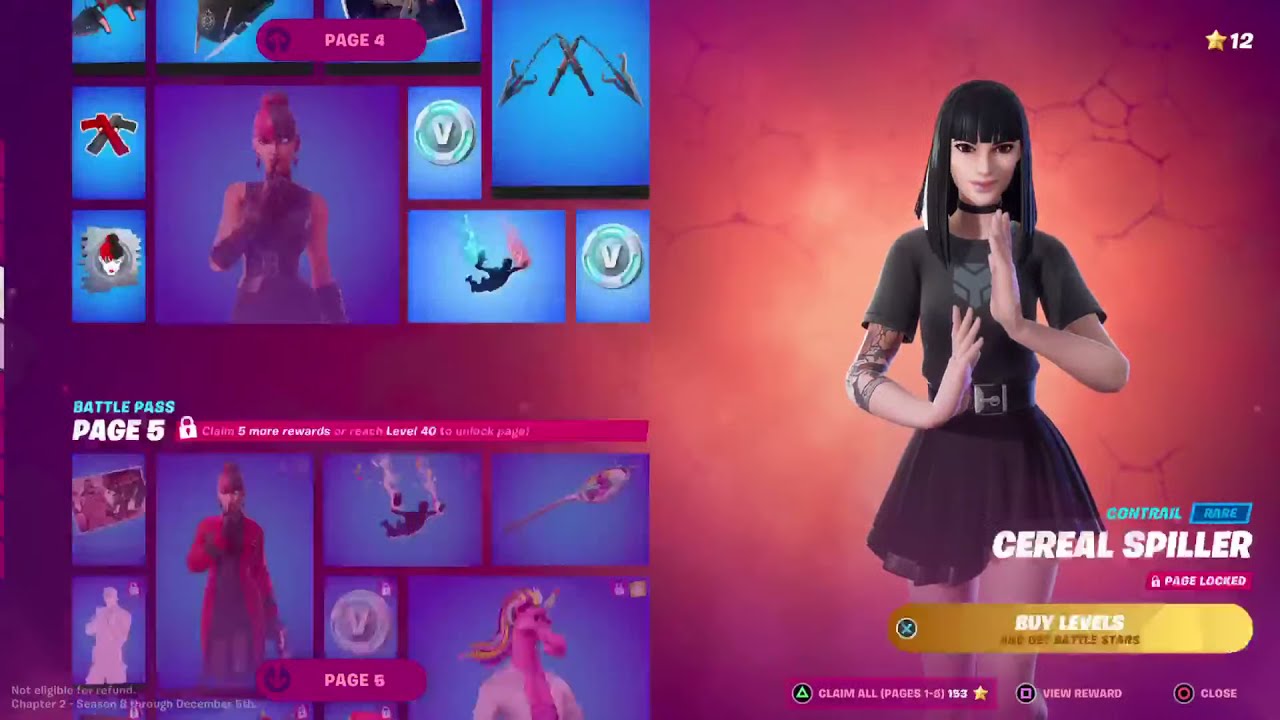The image features a detailed illustration of an animated character prominently displayed on the right side. She has shoulder-length black hair, dark eyes, and she is wearing a black dress with short sleeves, a short frilly skirt, and a belt around her waist. Notably, she has a tattoo on her right arm. The character appears to be in a dynamic pose with her hands held in front of her, palms facing each other, with one hand slightly higher than the other. The backdrop behind her is a vivid red and orange, reminiscent of the veins in a human heart.

In the lower right-hand corner of the image, there are various words such as "Serial Spiller," "Contrail," "Rare," "Page Locked," "Buy Levels," "Claim All," "View Reward," and "Close." Additionally, at the top right corner, there's a star symbol with the number 12 next to it, indicating some kind of ranking or level.

On the left side of the image, the background shifts to a purple hue with multiple blue square panels. These panels contain various icons and images, including pictures of tools, weapons, a pink horse wearing a white shirt, and several other characters. The image is rich with visual details and text elements typical for a video game interface, suggesting that it might be representing a character selection or upgrade screen within a game.